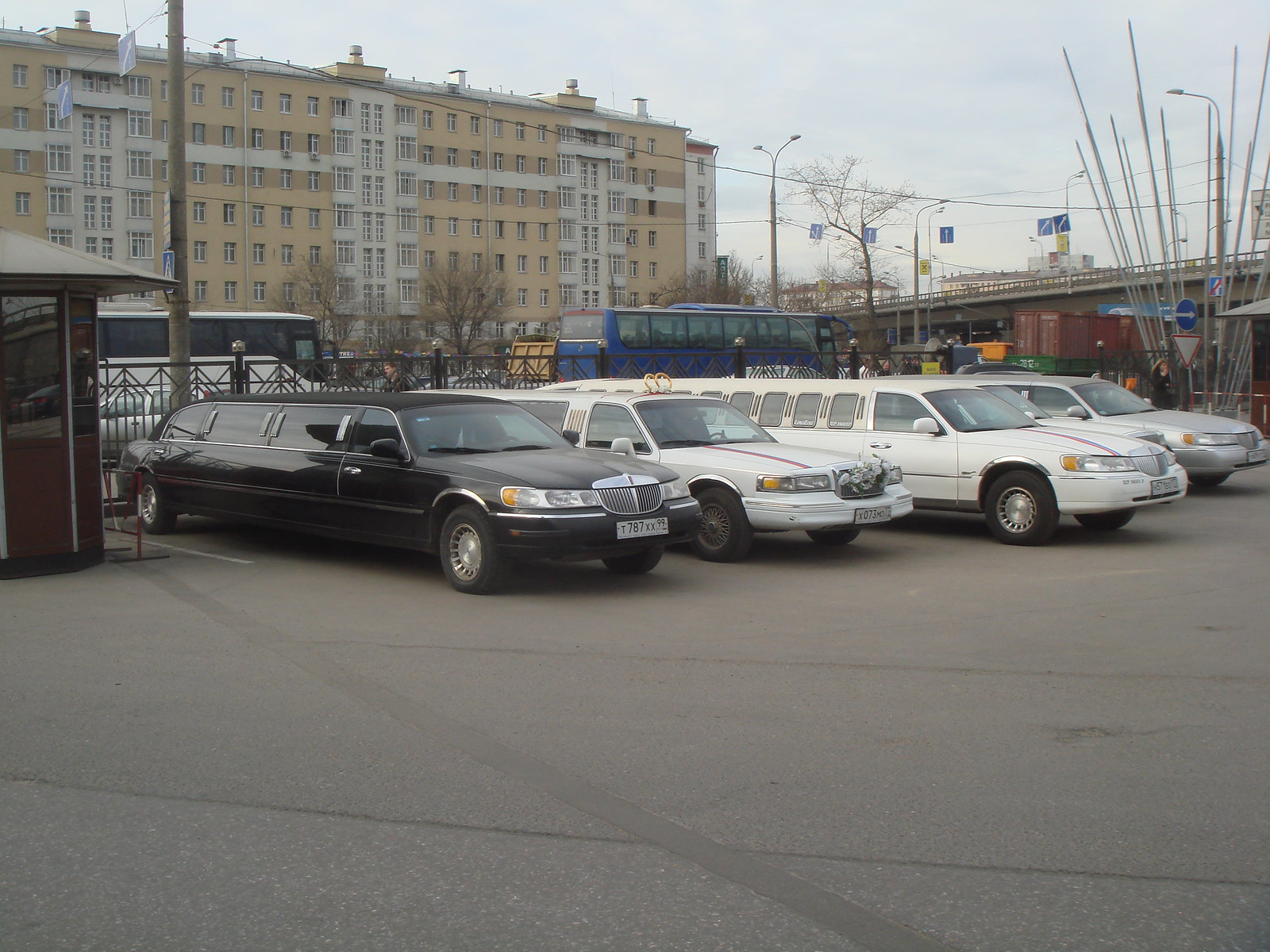The photograph captures a group of four long limousines, parked side by side in a car park on a cloudy but bright day. The limousines, each featuring multiple windows, include a black one, two white ones, and a silver one positioned on the right. The setting appears to be a busy city, evident from the presence of both a blue and a white bus in the background, along with various road signs and lamp posts. Dominating the background is a large, high-rise building with numerous windows, characterized by a yellow hue with pale whitish-yellow streaks. Nearby, there are bare trees and a road overpass, while the sky above is filled with dense clouds, hinting at a close-to-afternoon time. A spiky grey statue can also be noticed within the parking lot, adding to the urban landscape.